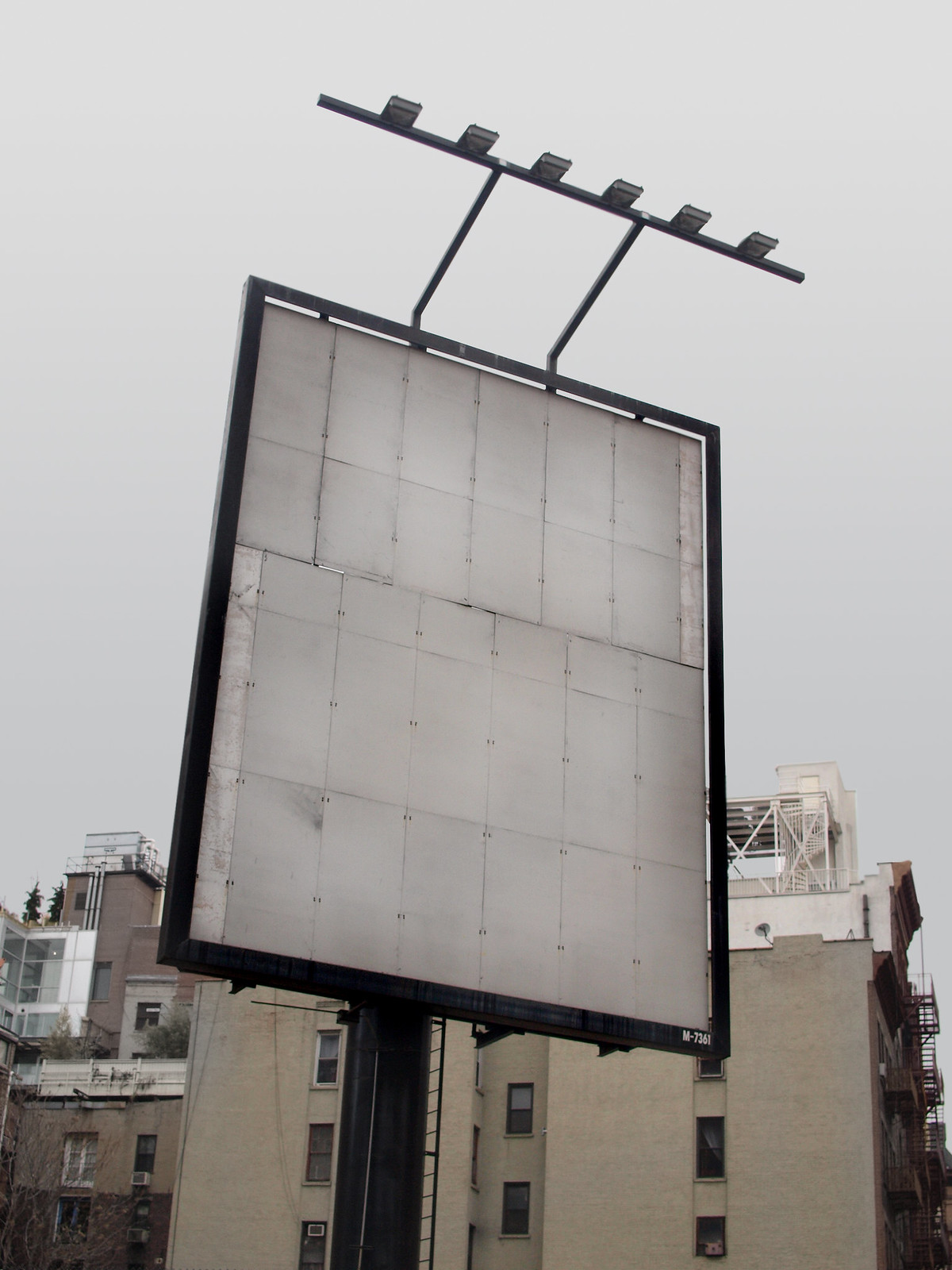In the foreground, a blank signage device stands prominently, framed in black and mounted on a sturdy black pole. This setup includes a ladder-like structure extending upward towards the sign. The sign itself is gray and features several rectangular slots, which are likely meant for placing signage inserts. At the top of the device, two black arms extend towards the camera, each topped with black squares that appear to be lighting fixtures designed to illuminate the signage below. In the background, multiple buildings with numerous windows are visible, set against an overcast sky with thick clouds obscuring direct sunlight. The setting suggests an industrial area.